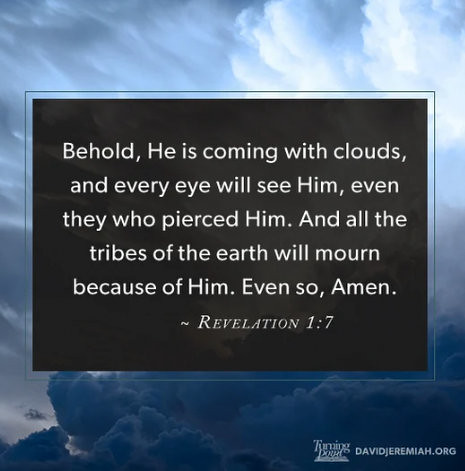The image depicts a poster with a background of fluffy, blue-hued clouds, giving it a serene and airy atmosphere. Overlaying this cloudy backdrop is a rectangular black card bordered in black. The card features a biblical quote in uniform white lettering that reads: "Behold, he is coming with clouds, and every eye will see him, even they who pierced him, and all the tribes of the earth will mourn because of him. Even so, Amen. Revelation 1:7." In the bottom right corner of the poster, the text "Turning Point, DavidJeremiah.org" is also written in white.